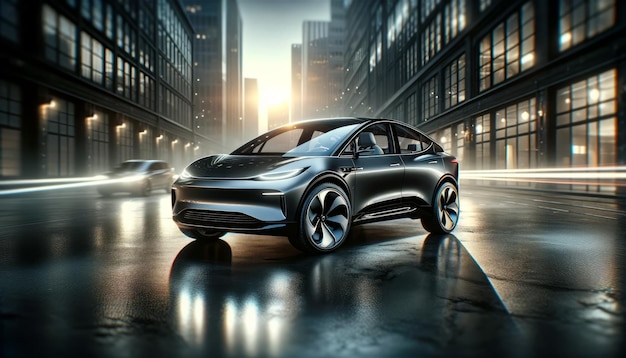The image showcases a sleek car, potentially a Tesla, prominently centered and facing diagonally on a street. The painting, rendered in blacks, grays, whites, and touches of light blue, especially highlighting the car, evokes a modern, almost digital aesthetic. The car's reflective surface hints at the street's polished ground, while a smaller vehicle with its headlights shining is visible in the background to the left. Towering buildings flank both sides of the street, their numerous windows either brightly illuminated or reflecting the surroundings. The right building displays more internal light, contrasting with the reflections on the left building. In the distant background, the setting sun casts a gentle glow, silhouetted by far-off skyscrapers, suggesting the onset of evening.